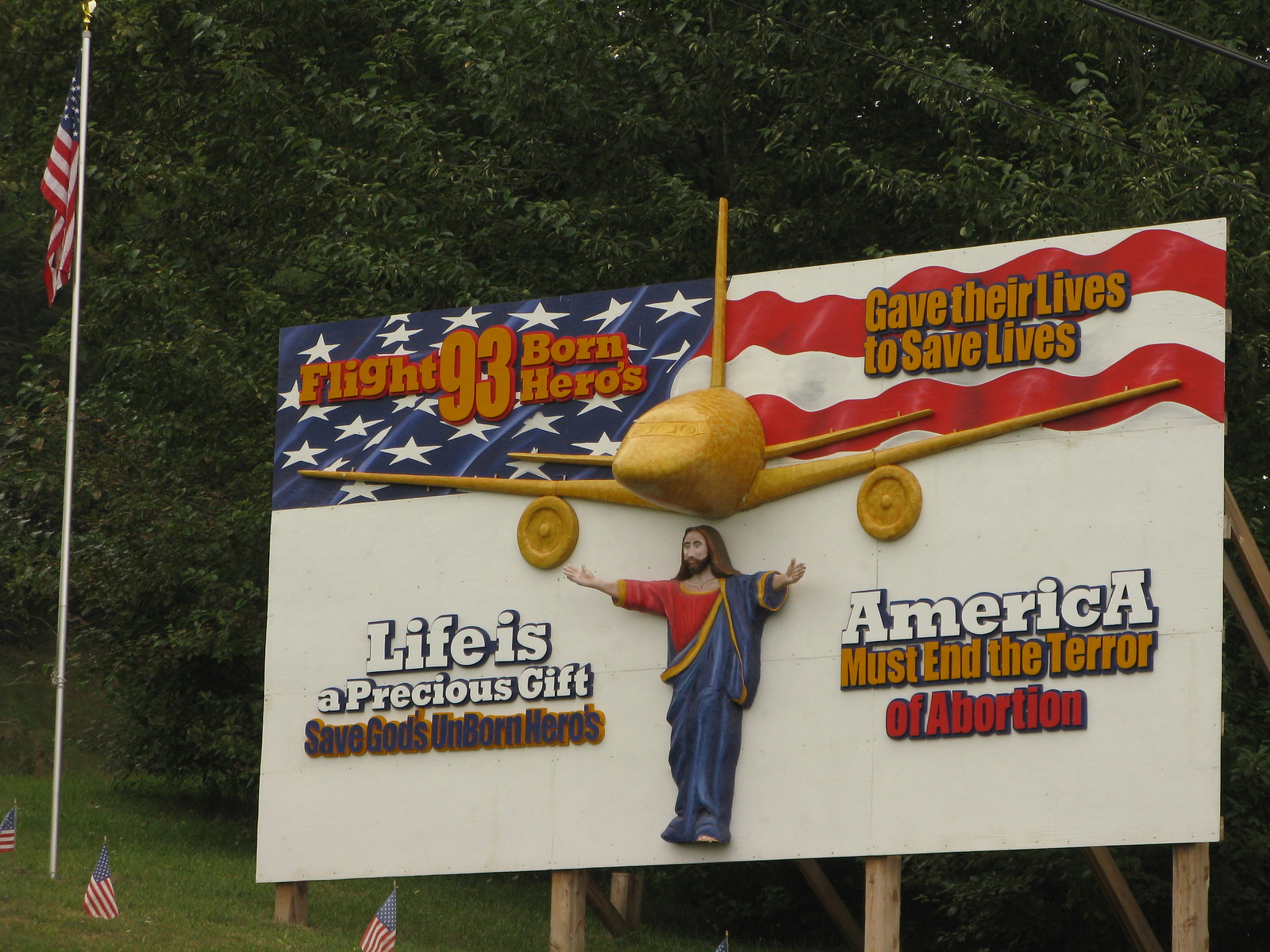In this rural setting, a large billboard features a striking image of Jesus with arms outstretched, adorned in a blue cape and red shirt, against a clean white background. The billboard's design is a blend of patriotic and religious imagery, starting with a depiction of the U.S. flag occupying the upper left corner—white stars on a blue background followed by red and white stripes. Bold yellow letters display the phrase "Flight 93, Born Heroes," honoring the heroes of the 9/11 attack. Below this, gold and yellow text reads "Gave Their Lives to Save," followed by another line in white letters with blue trim stating "America."

The message continues with a rallying cry displayed in yellow letters with blue trim: "Must End the Terror of," followed by red letters bordered in blue spelling "abortion." To the left, contrasting with the patriotic banner, another poignant message in blue trimmed white letters reads "Life is a Precious Gift," which is further elaborated below in yellow trimmed blue letters as "Save God's Unborn Heroes." An illustrative gold airplane is positioned just above the image of Jesus, linking the heavenly theme with the heroic Flight 93.

In the background, a tall tree with full green foliage suggests a summer timeframe. To the left of the billboard, a large U.S. flag flies high on a tall pole, accompanied by several smaller U.S. flags beneath it, heightening the patriotic atmosphere. This intricate scene masterfully intertwines themes of faith, heroism, and national pride.